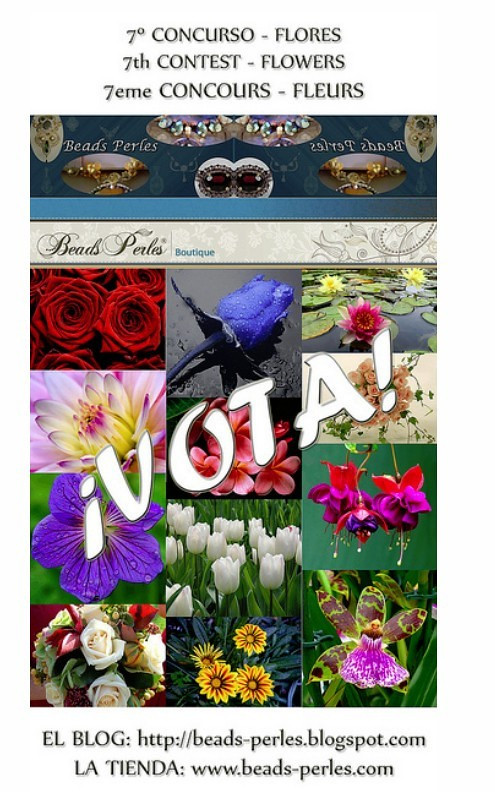The image appears to be an advertisement for the "70 Concurso Flores," which translates to the "70th Flower Contest," displayed in three languages: Spanish, English, and French. The top line in black, slightly blurred font reads "70 Concurso Flores" (Spanish), "7 Contest Flowers" (English), and "70 Concours Fleurs" (French). Below this, a captivating collage showcases various vibrant flowers and plants—red roses, purple blossoms, white tulips, yellow sun-like flowers, green shoots, purple rose-like flowers, and lily pads adorned with yellow and pink flowers.

A prominent banner at the top says "Beads Perles Boutique," indicating the shop's name. The words "Vota" (Vote) with an upside-down exclamation point, add a call to action on the left side. At the bottom, the advertisement features two website links in black: "El Blog" pointing to beads-pearls.blogspot.com and "La Tienda" directing to www.beads-pearls.com, presumably for more information and online shopping.